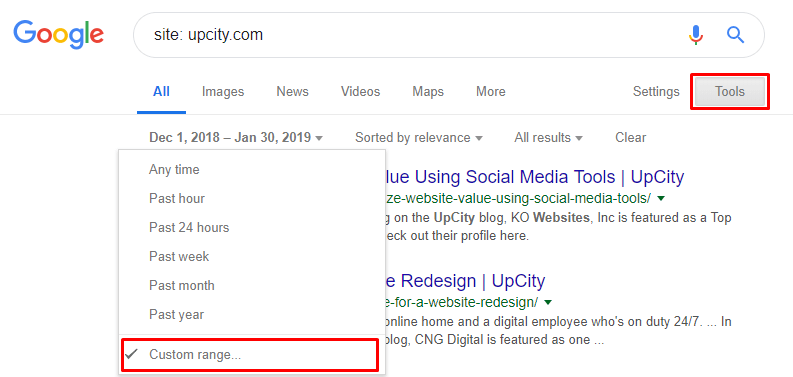The screenshot depicts the Google app interface on a computer screen. In the Google search bar, the query "site:appcity.com" is typed in black text. To the right of the search bar, there is a blue microphone icon adorned with Google’s iconic colors, alongside the standard search icon. Below the search bar, the "All" tab is selected and highlighted in blue, indicating that it is currently active. Beneath this, there is a date filter displaying the range from December 1, 2018, to January 30, 2019. The filter appears as a pop-up with options—the word "Tools" is highlighted in a red box with green text, signifying it has been clicked. Additionally, a "Custom range" option is also within a red box. The search results on the page feature links primarily colored in blue, accompanied by supplementary text in black, green, and gray.